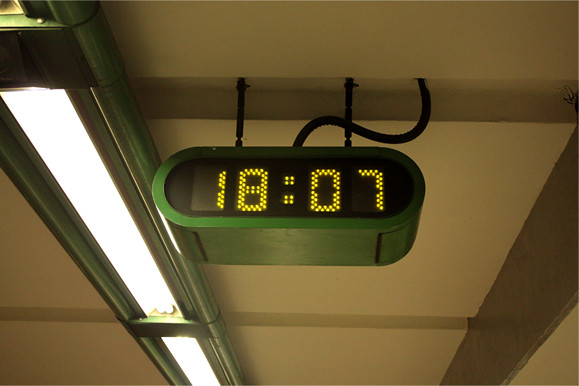This is a colorful image of an oval-shaped, kelly green digital clock that is prominently hanging from a white, square-brick ceiling via two short black metal pieces attached at the bottom. The clock displays the time "1807" in yellow LED digits on a black background. A distinct black wire curves from the middle of the clock up into the ceiling, likely serving as a power supply. Directly to the left of the clock is a green (olive/kind of green) metal fluorescent light fixture, revealing its light bulbs inside. The top of a gray wall is visible to the left. The ceiling also features some brown lines, and there may be a wood beam on the right side, adding to the structural complexity of the scene.